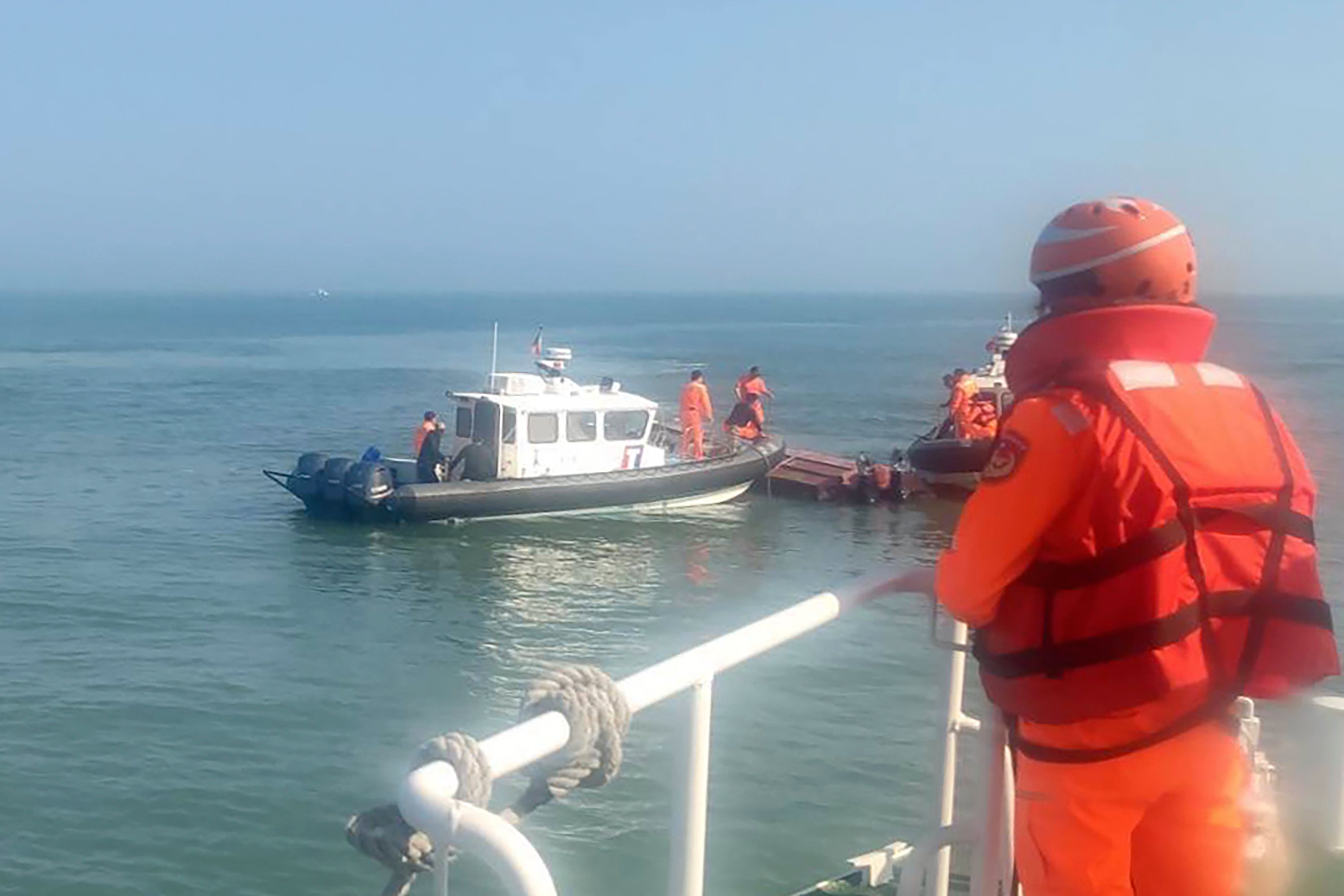In this slightly hazy photograph, possibly due to fog or low resolution, a serene backdrop of blue sky and expansive blue water sets the scene. In the foreground, a person clad in high-visibility orange gear, including an orange helmet with white stripes and an orange jacket with an attached life vest, stands on a white-metal-bar-fenced platform, likely part of a boat or pier. The individual’s light orange pants complete the outfit, and a cream-colored rope is tangled around the railing nearby. 

This individual is gazing out at a white tugboat with black lining and three motors at the back, which reflects slightly in the water. The tugboat carries about six or seven crew members, all similarly dressed in vivid orange gear. The crew appears to be managing or hauling floating logs or metal tubes. High overhead, an American flag flutters, adding a touch of color and patriotism to the maritime scene.